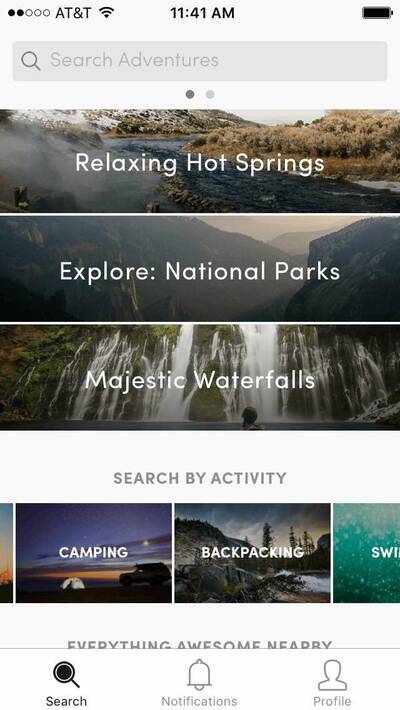This screenshot, taken from a cell phone, features the AT&T service provider at the top with two out of five bars of signal strength and full Wi-Fi connectivity. The time displayed is 11:41 AM, and the battery icon shows it's fully charged. Below this information, there's a menu bar including a grayed-out search field labeled "Search adventures," accompanied by a search icon. Two dots underneath indicate the ability to swipe between pages.

The main content showcases various travel themes: "Relaxing Hot Springs," with an image of a soothing hot spring; "Explore National Parks," featuring a picturesque mountain scene; and "Majestic Waterfalls," highlighted by a captivating waterfall image, partially obscured by someone's head in the lower portion of the screen. Following this visual display, there's a white gap with the text "Search by activity," leading to a slideable menu showing categories such as "Camping," with an image of a tent under a night sky; "Backpacking," displaying a scenic landscape; and a partially visible category starting with "SWI," likely indicating "Swimming."

Further down, partially cut-off text reads "Everything awesome nearby," followed by another menu bar where the "Search" option is highlighted, alongside unselected options for "Notifications" and "Profile." The overall impression suggests that this screenshot is from a travel app, focused on the search menu where users can explore various vacation options.